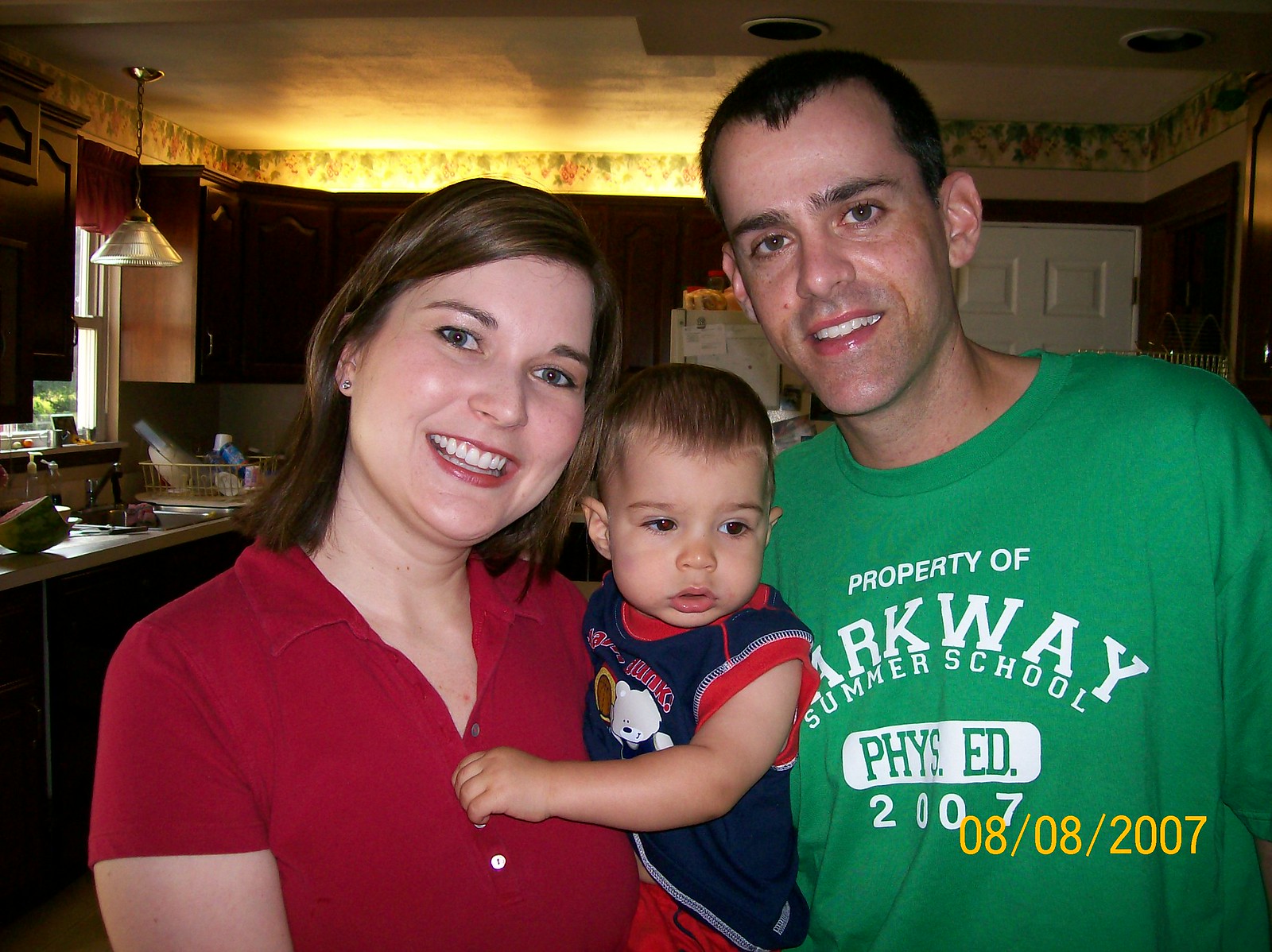In this detailed family portrait taken indoors on August 8th, 2007, a husband and wife stand in their kitchen holding their young toddler. The mother, wearing a short-sleeve red polo shirt, has short brown hair and blue eyes and stands smiling on the left. The father, positioned to the right, wears a green t-shirt with the words "Property of Parkway Summer School Physical Education, 2007" and has dark hair and eyes. The toddler, with blondish-brown hair and dark eyes, is cradled in the mother's arms, dressed in a sleeveless red and blue shirt with matching red shorts. Though the child appears a bit confused and looks away from the camera, the parents smile warmly. The background reveals typical kitchen details, including cabinets, a sink, dish drain, faucet, and a window letting in natural light from the left. A white door is visible to the right. The image has a yellow watermark on the bottom right corner.